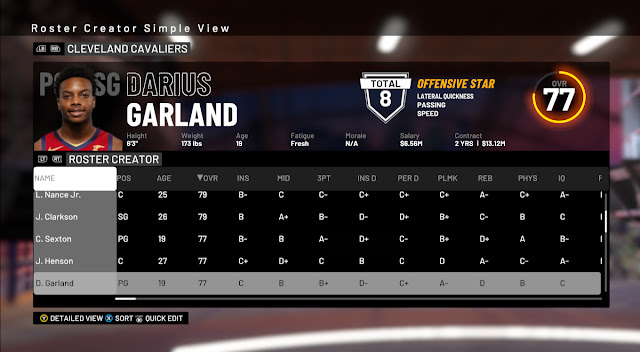The image appears to be a screenshot of a sports management or roster creation software on a computer. The background at the top is predominantly black, showcasing options such as 'Roster Creator' and a 'Simple View'. Below this header, the name 'Cleveland Cavaliers' is prominently displayed, possibly indicating the team being managed. Three indicator lights stretch across this section.

Beneath this, there's a gray area featuring a player's profile. The player, identified as Darius Garland, is an African American wearing a red tank top adorned with a Nike swoosh on the left side. Adjacent to his image, 'Darius Garland' is clearly stated. To his right, a shield icon displaying the number '8' is visible, along with yellow text listing attributes like 'Offensive Star', 'Lateral Quickness', and 'Passing Speed'. A yellow circle embossed with the number '77' seems to be indicative of a rating or performance metric.

Below the player profile, the 'Roster Creator' feature reappears, complemented by a vertically aligned menu showcasing player names. The list includes L. Nance Jr., A. Clarkson, C. Sexton, J. Henson, with Darius Garland being the last, highlighted within a gray border. The section provides various ratings across the screen for these players.

In the lower-left corner of the image, options for 'Detailed View', 'Quick Sort', and 'Quick Edit' are visible, likely tools for further interaction or analysis within the software.